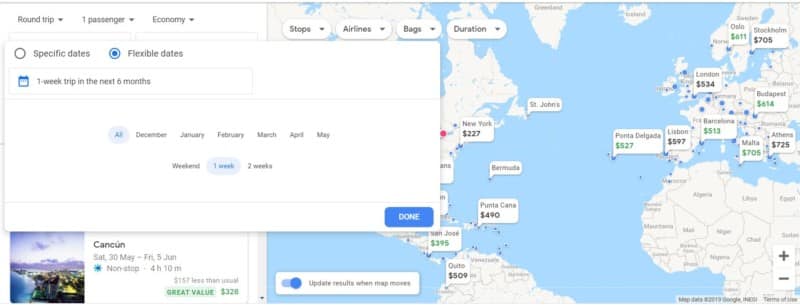The image is a detailed screen capture of a vacation planning website, specifically focusing on flight options. The primary feature displayed is a detailed map overlay showing various prices for flights to different destinations. To the left, a horizontal menu presents options for configuring the search, including "Round-trip," "One Passenger," and "Economy."

A pop-up box on the left side of the screen allows for date customizations. The top left of this box provides options for "Specific Dates" and "Flexible Dates," with "Flexible Dates" currently selected. Beneath this selection, the text specifies a "One week trip in the next six months." 

Further down, months from December to May are displayed, with all months selected. Additional trip duration options—"Weekend," "One week," and "Two weeks"—are listed, and "One week" is chosen.

In the lower right corner of the pop-up box, a visible button likely finalizes the date selection. Just beneath the pop-up, partially obscured, is information hinting at a sample destination and date: "Cancun," with a flight planned for "Saturday, May 30th." The image also features clickable elements for "Stops," "Airlines," "Bags," and "Duration," likely for further flight search refinement.